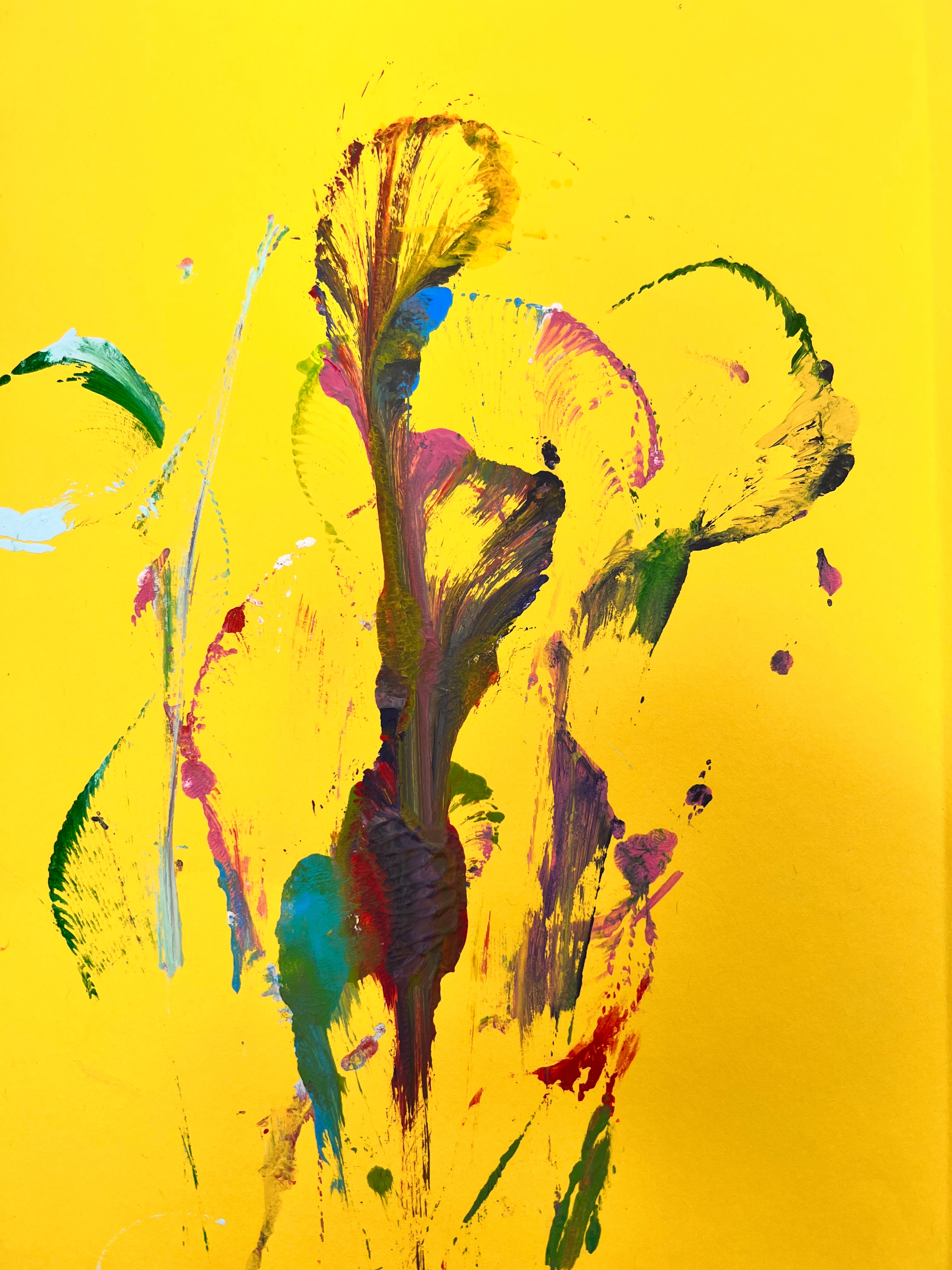This vibrant abstract painting features a striking yellow background, reminiscent of a canvas bathed in bright sunlight. The composition is a rectangular form presented on a vertical slant, filled with an array of dynamic and contrasting paint streaks and smears. The central area of the piece is dominated by a chaotic blend of colors—green, blue, pink, yellow, purple, and aqua—culminating into a sickly brown smear that anchors the artwork.

Prominent among the brushstrokes is a long burgundy line that travels vertically and fans out into a petal shape, incorporating semi-circular formations of pink and dark green. To the left, a distinct green stroke amidst white splodges and streaks provides texture, while to the right, purple, pink, and brown paint merge into an inverted guitar-like shape. These colors and shapes trickle downward across the canvas, leading towards a focal point at the bottom characterized by mingling red, green, and yellow hues.

Thick paint layers create varying textures throughout, giving the impression of a haphazard, yet deliberate, artistic experimentation. The entire piece appears as though it captures the spontaneous, energetic movements of the artist, perhaps even resembling a scanned image in its detailed, high-contrast presentation.